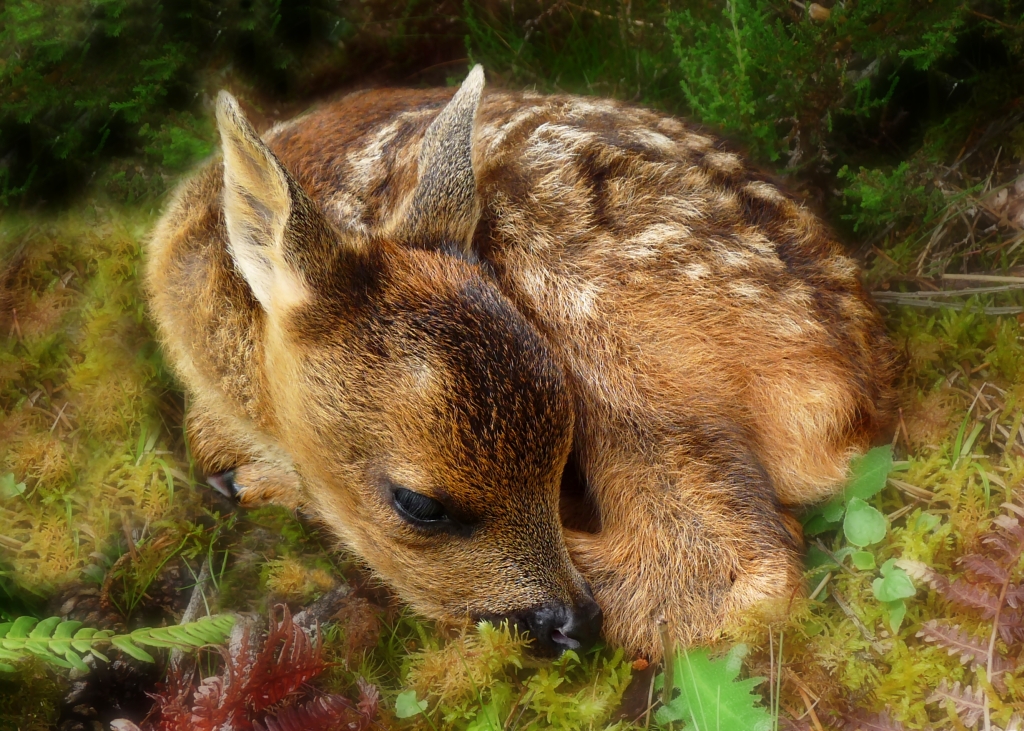In this detailed photographic image, we see a peaceful, young fawn nestled at the center of an outdoor forest setting during the daytime. The fawn, with its light to dark brown fur adorned with white spots, is curled up with its head nestled near its tail. Its legs and tail are tucked beneath its body, creating a compact, restful pose. The fawn's large, black eyes are open but gazing downward, and its pointy ears catch patches of sunlight filtering through the trees.

In the foreground, a mix of green leaves, red leaves, and yellow grass can be seen, adding to the natural, serene atmosphere of the scene. The animal's fur appears very clean, and the play of light and shadow gives the image a tranquil ambiance. Darker areas of the background lead into green bushes and possibly evergreen shrubs, creating a lush setting. The sunlight dapples both the fawn and the surrounding forest floor, casting a warm glow over the peaceful tableau.